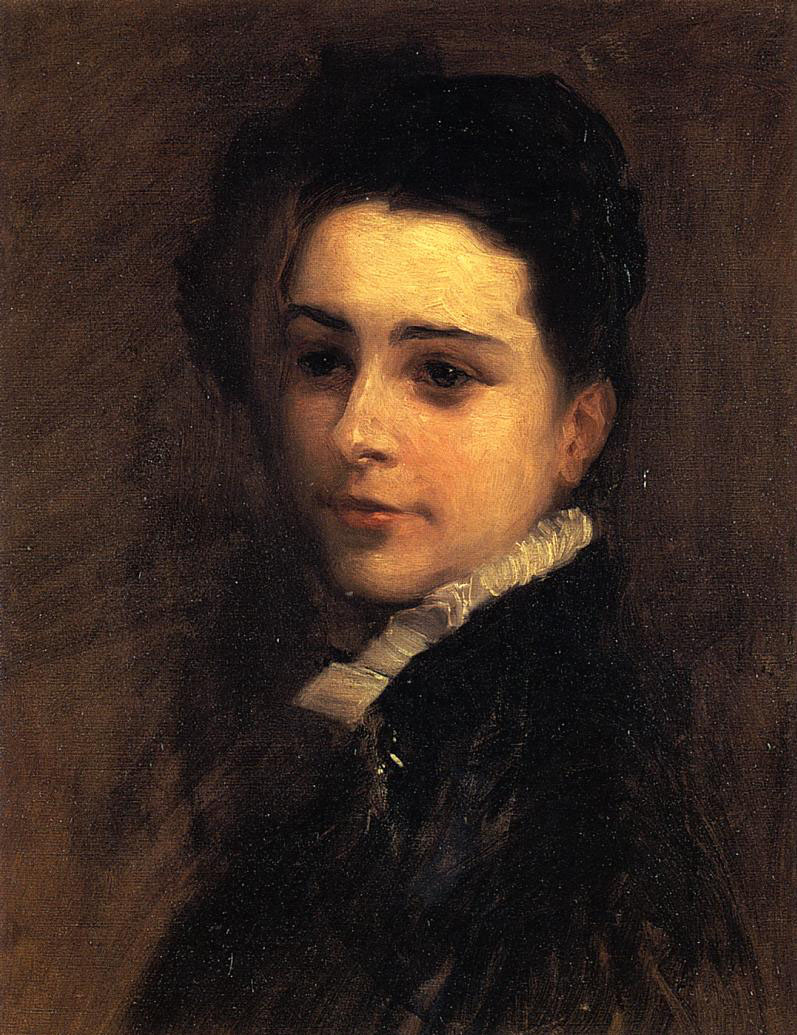This is a dramatic, vertically-oriented portrait painting reminiscent of the Renaissance style, evoking techniques possibly akin to those of Rembrandt. The subject appears to be a young person, likely a woman, with her hair tied up and possibly wearing a black cap or bonnet. She is turned sideways, looking over her left shoulder toward the viewer, with a serious yet gentle expression highlighted by large, dark brown eyes and dark eyebrows. Her face, illuminated with soft white undertones and detailed with hints of brown, features a small mouth and a petite nose. The subject is donned in a dark black coat accented by a distinctive white ruffled or frilly collar, rendered with bold brush strokes. The background is a sombre dark brown, interspersed with subtle brush strokes, creating a stark contrast that draws focus to the smoothly painted, radiant face, which is the brightest element in the composition. The lower part of her form blends into an abstract, black area with white highlights, executed in an undefined manner that enhances the overall mysterious and striking visual impact of the piece.